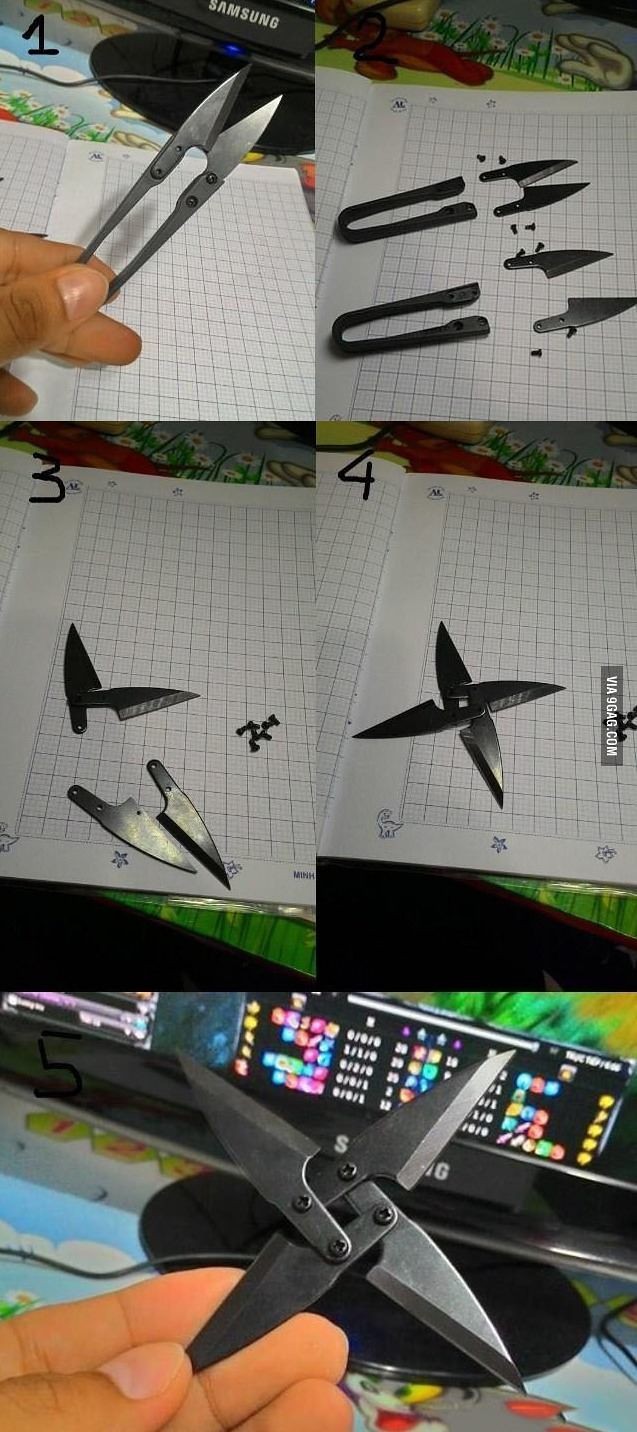This vertically cropped image is a step-by-step tutorial for assembling a metal throwing star. It is organized into five sections: the top two-thirds feature four equally-sized rectangular sections arranged vertically, while the bottom third consists of a larger rectangular section. Each of the top four sections illustrates a step in the assembly process, depicted on white graph paper. In step one, a hand is shown holding metal segments with fingers visible. Step two displays the screws and metal components necessary for assembly. Step three demonstrates how two segments are screwed together, and step four shows the assembly of two sets of these segments, forming a cross-shaped star. The bottom, larger section presents an up-close view of the finished product—a sharp-edged, black metal throwing star—held in the person's left hand. The image clearly highlights the sharpness of the blades, connected by visible screws with a central hole, illustrating the intricate assembly process and the final compact size that fits within a hand.